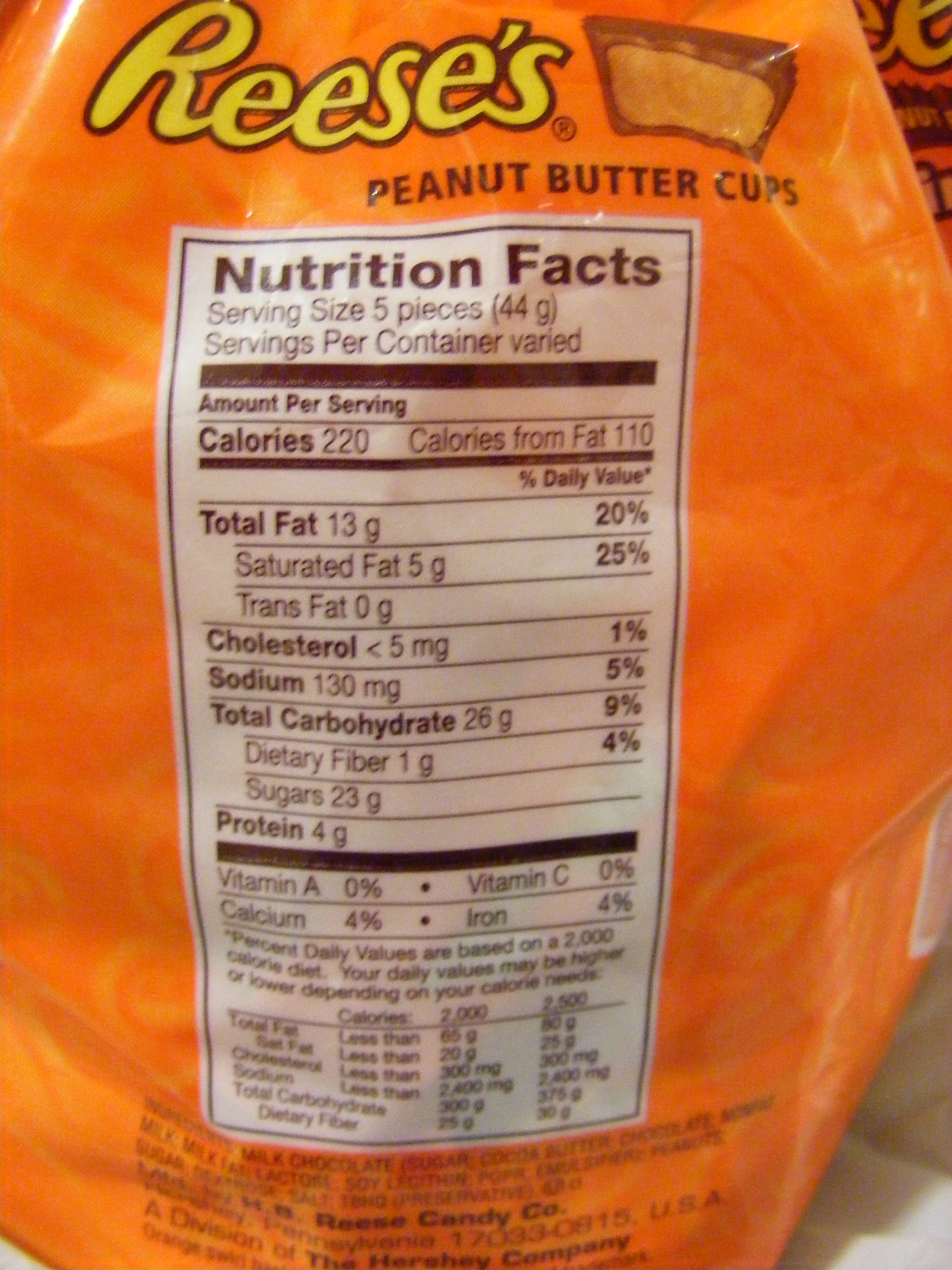This detailed color photograph captures the nutritional information displayed on the side of a bright orange Reese's Peanut Butter Cups bag. At the top, "Reese's" is emblazoned in yellow cursive font accompanied by a trademark symbol and a graphic of a peanut butter cup with a bite taken out of it. Below this, "peanut butter cups" is written in black. The image prominently features the nutritional facts label set against a white background, which reads "Nutrition Facts" in black.

The label specifies that the serving size is five pieces, totaling 44 grams, with servings per container varying. Each serving contains 220 calories, 110 of which are from fat. The total fat content per serving is 13 grams, which is 20% of the daily value. This includes 5 grams of saturated fat (25% of the daily value) and 0 grams of trans fat. The cholesterol content is less than 5 milligrams, constituting 1% of the daily value. The sodium content is 130 milligrams, equating to 5% of the daily value. Total carbohydrate content is documented at 26 grams (9% of the daily value), including 1 gram of dietary fiber (4% of the daily value) and 23 grams of sugars. Each serving provides 4 grams of protein. The presence of vitamins and minerals such as Vitamin A, Vitamin C, Calcium, and Iron are specified as follows: 0% Vitamin A, 0% Vitamin C, 4% Calcium, and 4% Iron. The label notes that these percent daily values are based on a 2,000 calorie diet, and individual daily values may vary. Additional smaller text concerning ingredients and other nutritional information appears at the bottom of the label but is noted to be blurry and difficult to read.